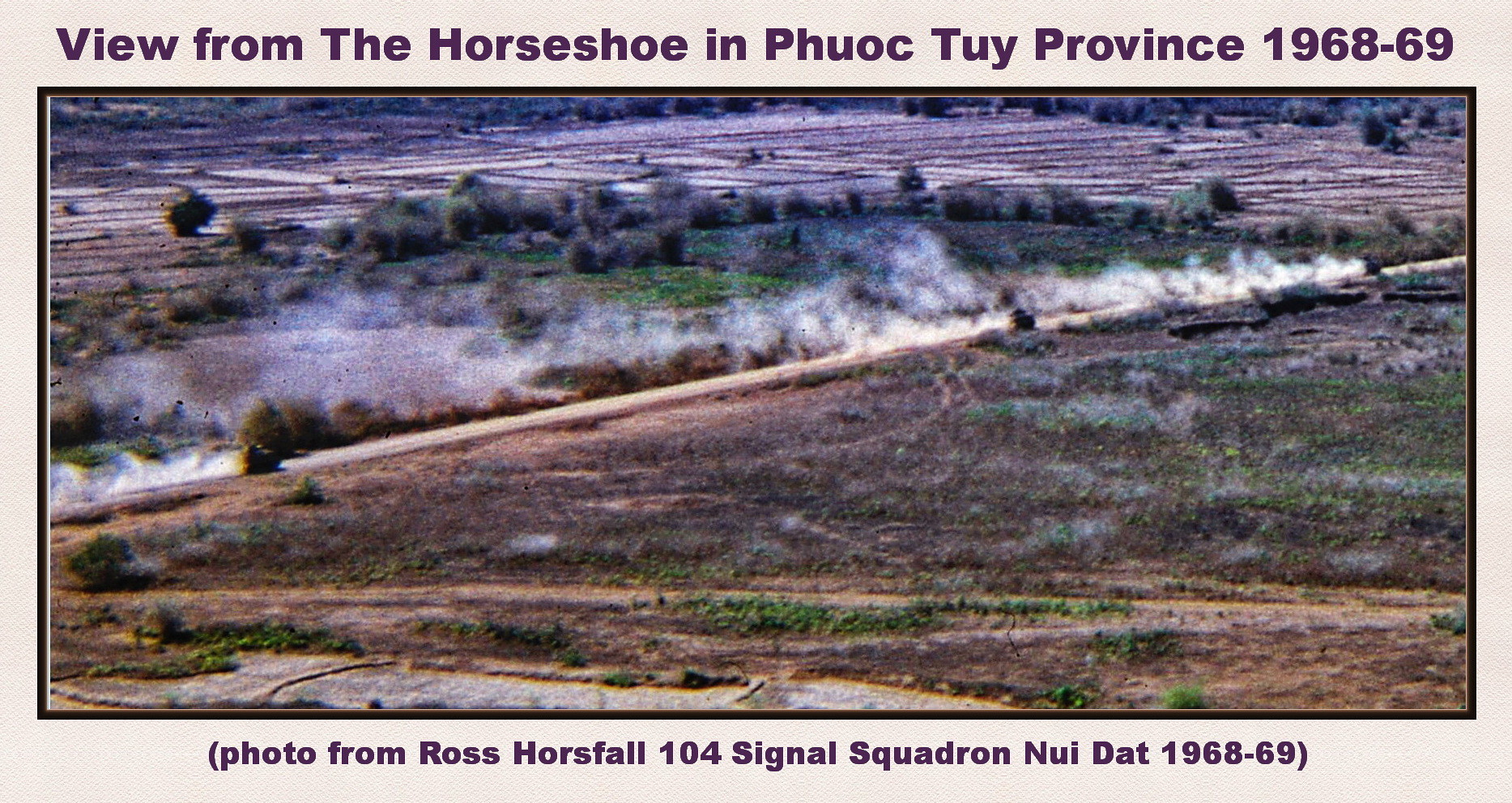This historical photograph captures a mist-covered trail that evokes the atmosphere of a locomotive steam track. The trail is surrounded by lush, grassy vegetation and dense weeds, adding to its rugged, untamed appearance. In the background, you can see a wide expanse of dirt lot extending beyond the trail. The top of the photograph is inscribed with the text: "View from the Horseshoe in Phuoc Thai Province 1968-69." The bottom of the photograph credits the image to Ross Horsefall of the 104 Signal Squadron, Nui Dot, during the same period. This suggests that the photograph was taken in Phuoc Thai Province, likely during the Vietnam War, highlighting a significant locale through the eyes of those who served there.